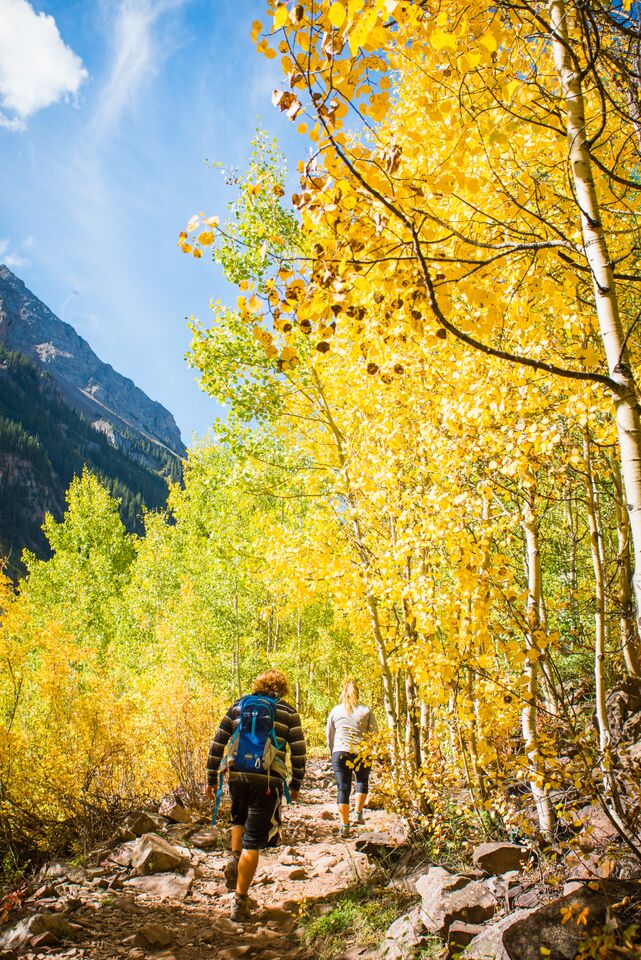This tall, rectangular photograph captures a serene daytime hike through a picturesque mountainous trail. In the bottom portion of the image, two hikers—a man and a woman—are walking away from the camera. The man, positioned slightly to the left, has red curly hair tied in a ponytail and is dressed in a long-sleeved striped shirt, dark knee-length shorts, hiking boots, and a blue backpack. Next to him, slightly ahead, the woman sports a blonde ponytail, a gray tight long-sleeved shirt, black leggings, and hiking shoes.

The trail, composed of light brown dirt and large gray rocks, meanders from the bottom left corner into the distance. To the right, a dense wooded area features very tall, thin trees with striking yellow leaves, while the background on the left showcases a different set of trees with lush green foliage. Extending towards the top left corner, the image reveals a distant mountain range under a clear blue sky dotted with wispy white clouds, and the mountain peaks appear to be dusted with snow. The ground around the trail is a mix of rocks and various vegetation, creating a vibrant scene of green, yellow, brown, and red hues—perfect for a refreshing hike.